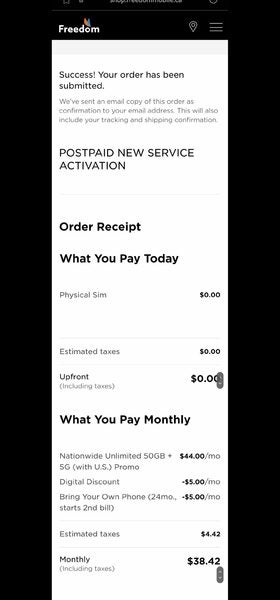In this image, we see a detailed order receipt from a company named "Freedom," indicated by a logo at the top left corner within a black-bordered section. The receipt contains a white area inside the black border that serves as an order summary screen. 

At the top of the white area, a message confirms the order's success: "Your order has been submitted. We've sent an email copy of this order as confirmation to your email address. This will also include your tracking and shipping confirmation." 

The receipt specifies that the order includes a "Postpaid new service activation" with no upfront costs (Physical SIM: $0, Estimated taxes: $0, Upfront: $0). 

It then outlines the monthly charges as follows:
- Nationwide Unlimited 50GB Plus 5G with US Promo: $44 per month
- Digital Discount: -$5 per month
- Bring Your Own Phone discount (24 months starting from the second bill): -$5 per month
- Estimated taxes: $4.42

The total monthly cost, including taxes, amounts to $38.42.